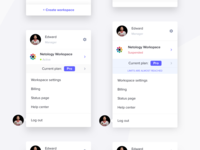The image is blurry, depicting six pages arranged in a grid. The top two pages are partially visible, showing only their bottom sections. Similarly, the bottom two pages reveal only their top sections. The two central pages are fully visible. All the text on these pages is in Braille, making it unreadable due to the blurriness. 

Each page contains both black and white text, with black text primarily on the top and a white text overlay on a blue background button, likely for selecting an option to proceed. The backdrop of these pages is light gray, providing a contrast to the white pages. 

Each page also features a profile picture or page icon in the top-left corner, which is circular and shows an individual wearing white and red attire. The same profile icon is repeated at the bottom-left corner outside of the pages as well. The overall image is defined by its blurriness, making detailed text and smaller features difficult to decipher.